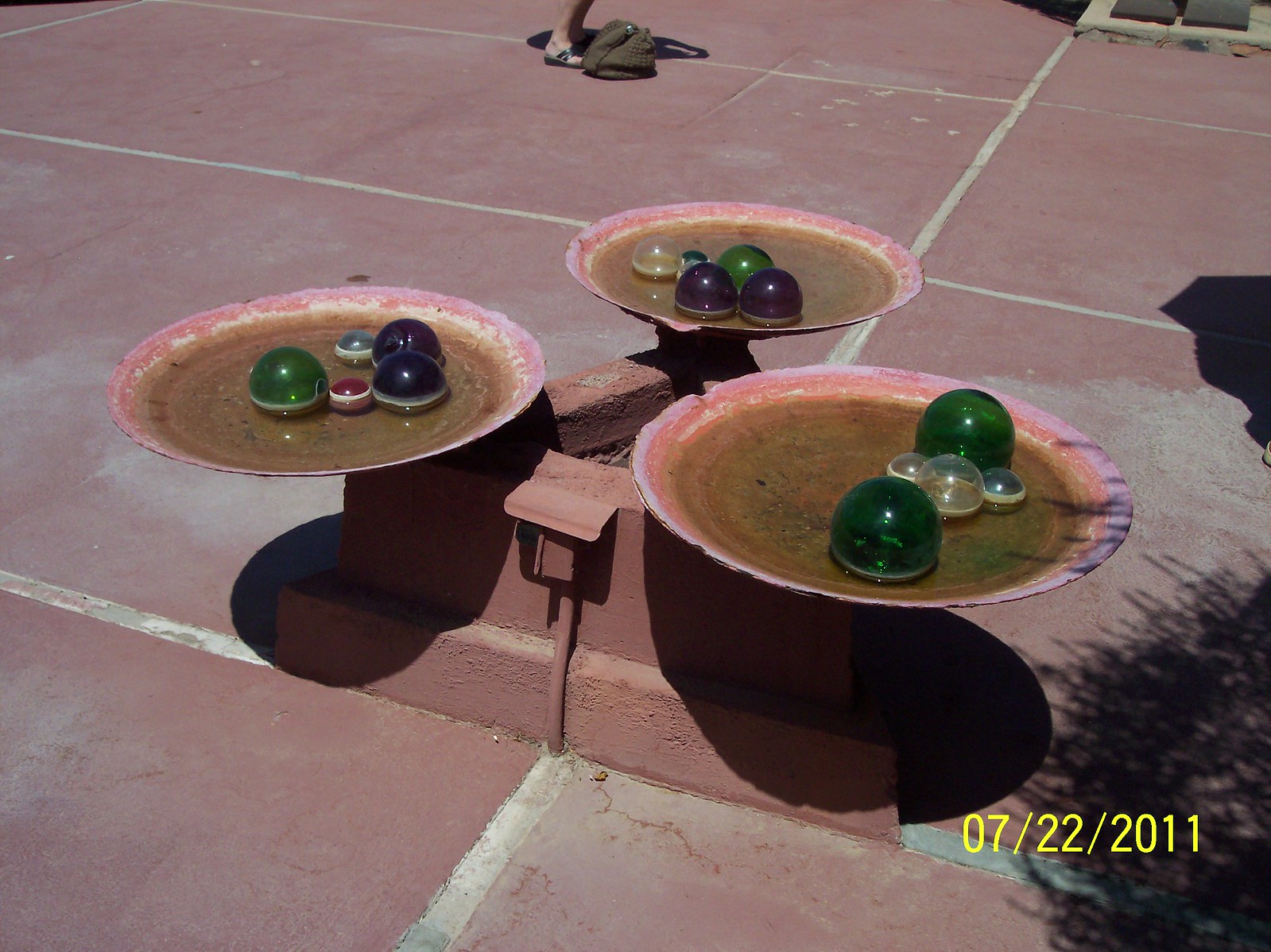The image captures an outdoor art display set on a reddish, concrete-like ground with large rectangular white lines. At the center, there is an open V-shaped triangular platform made of what appears to be a blend of concrete and clay materials. At each point of this V-shaped structure, there are round, shallow water basins resembling birdbaths, slightly weathered with a rusty look, containing dirty water. Each basin is adorned with various orb-shaped decorative objects in colors ranging from green, white, purple, blue, pink, and red. These orbs vary in size and include both translucent and solid hues, floating or resting within the water.

In the background, a partial view of a person wearing black sandals can be seen, along with a small portion of a green or brown cloth bag near their feet. Also visible is the shadow of foliage and a small bush protruding from the edge of the display. The image is dated in yellow at the bottom right corner, reading 07/22/2011.